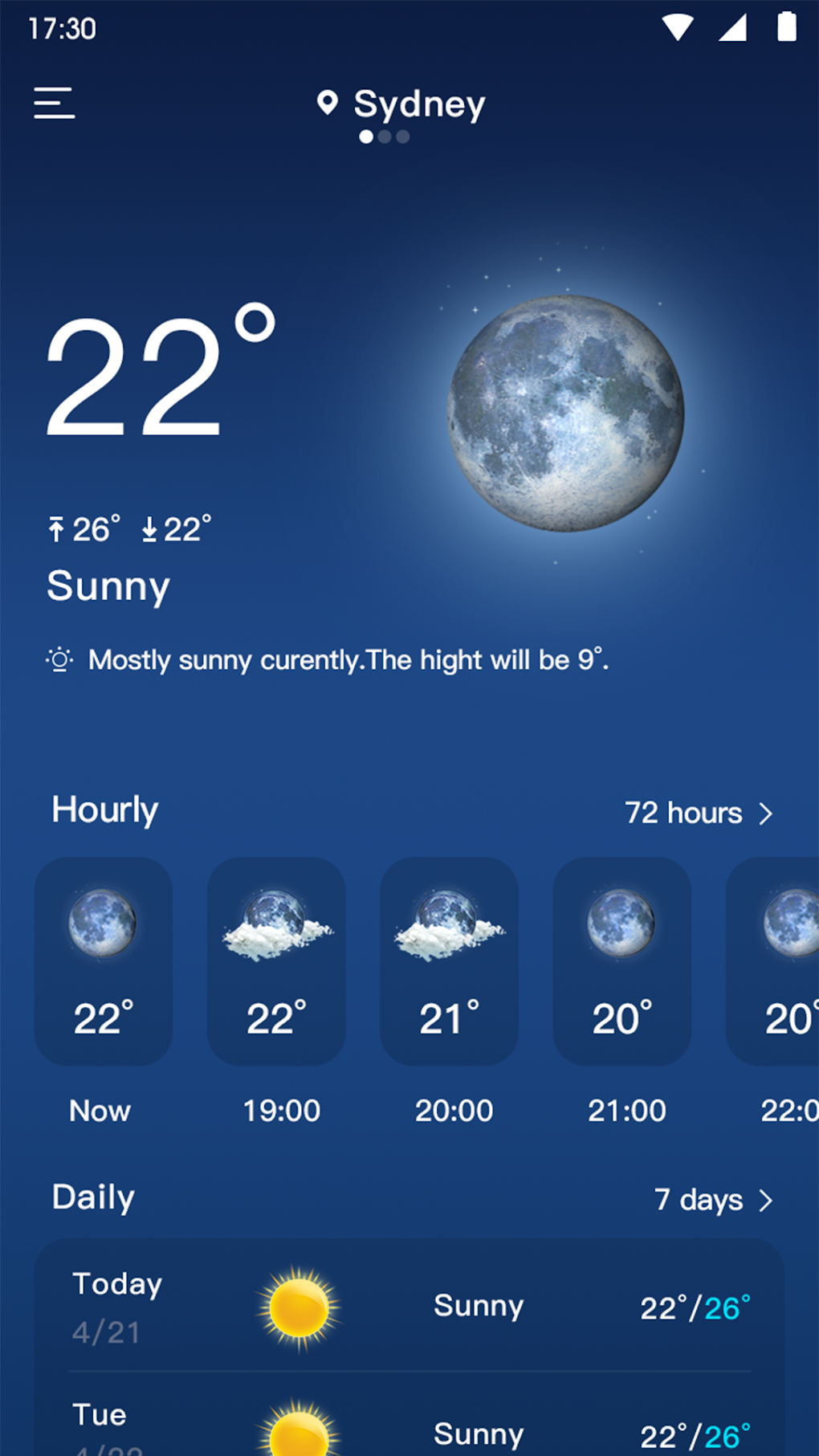The screenshot depicts a cell phone displaying a weather forecast interface. At the very top, the time reads 17:30, followed by icons representing a full internet signal, strong connectivity bars, and a fully charged battery, all in solid white. Below this, the header "Sydney" is positioned above a weather summary.

Directly beneath these elements, the temperature is shown as 22 degrees Celsius with a degree symbol, accompanied by an icon of the Earth. The current weather condition is described as "Sunny" with detailed temperature readings of a high of 26 degrees and a low of 22 degrees.

Continuing down, the forecast describes the weather as "Mostly Sunny" with a high of 9 degrees (likely based on a different time or location). Below this, the "Hourly" section includes several icons representing the Earth with varying cloud cover and corresponding temperatures: 22 degrees, another with clouds at 22 degrees, 21 degrees, and two icons at 20 degrees.

Further down, under the "Daily" section, a seven-day weather forecast begins with "Today" featuring a sun icon, indicating sunny weather with temperatures between 22 and 26 degrees. The subsequent day, Tuesday, repeats the sunny forecast with identical temperatures of 22 and 26 degrees.